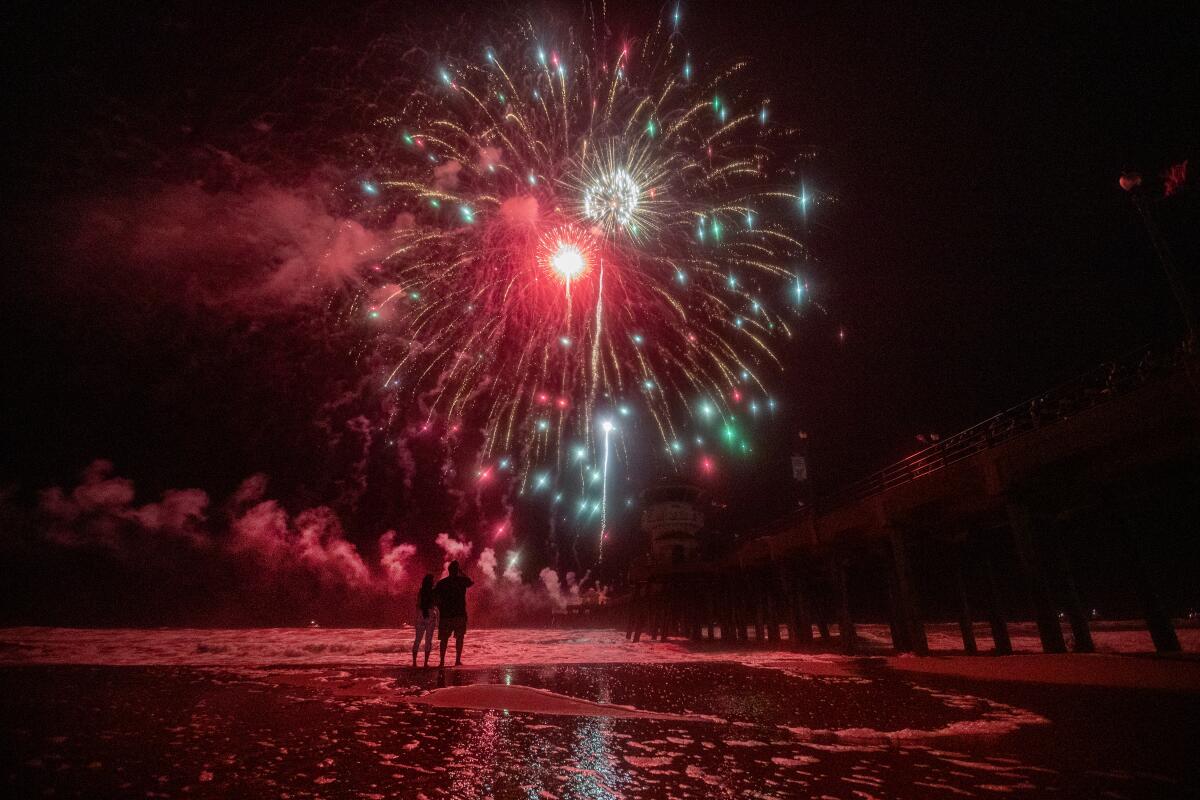This photograph, set outdoors on a beach at night, captures a couple standing at the water's edge, looking up at a vibrant display of fireworks. Both the woman, with long black hair, and the slightly overweight man are dressed in shorts, their backs turned to the camera, and are positioned slightly off-center, leaving a view of the surrounding scene. The night sky, dark and expansive, is illuminated by two prominent fireworks bursts—one a yellow ball, the other white, with protruding sparks. The colors in the fireworks are predominantly orange but also include hues of red, green, pink, fuchsia, blue, and white, casting a colorful glow over the scene. Faint dusky pink and gray smoke trails from the explosions. To the right side of the couple, a long boardwalk on piers extends over the water, leading to a tower at its end. The fireworks occupy about a third of the image, providing the primary illumination against the otherwise dark backdrop, emphasizing the couple's serene silhouette framed by the beach and ocean. The image, absent of any text, demonstrates professional quality and a clear, detailed capture of the moment.